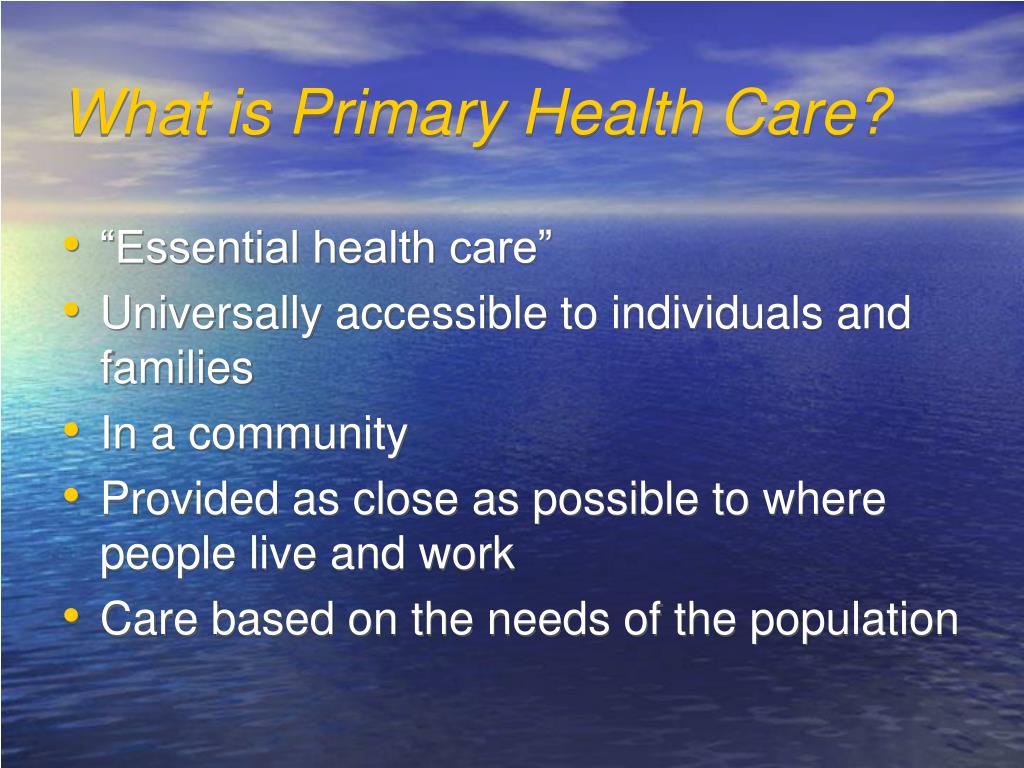This is a descriptive slide featuring the question "What is primary health care?" in yellow text as a bold heading at the top. The slide is set against a serene background image of a blue sea meeting a blue sky, with light shining brightly from the left side, illuminating the water. Beneath the heading, there are five informational bullet points, each with yellow bullet markers and white text. The points highlight core aspects of primary health care: "essential health care," "universally accessible to individuals and families," "in a community," "provided as close as possible to where people live and work," and "care based on the needs of the population." The overall design combines the tranquility of the ocean scene with clear, vital information on primary health care principles.